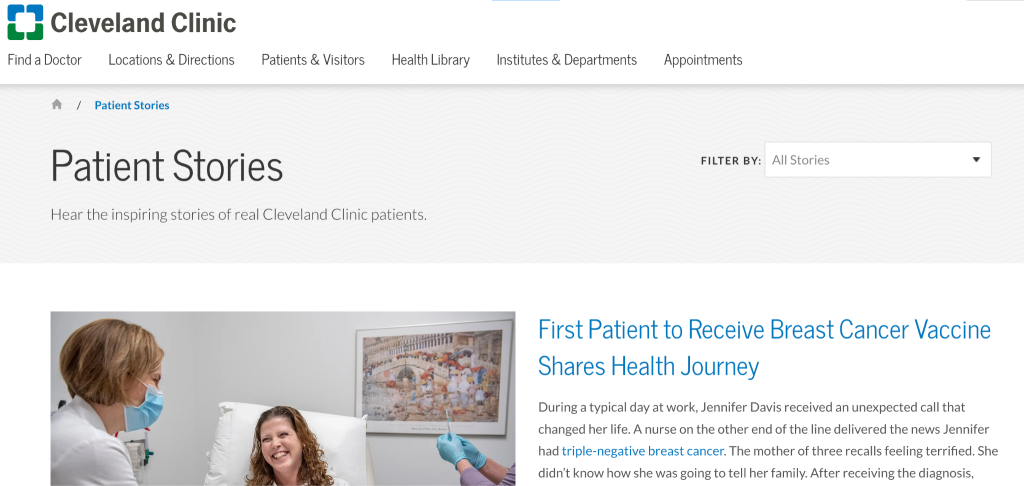Caption: 

The homepage of the Cleveland Clinic website is displayed with a gray background. At the top left, the Cleveland Clinic logo is prominently featured. Central to the page is an inspiring section titled "Patient Stories," inviting visitors to "Hear the inspiring stories of real Cleveland Clinic patients." Below the title, there's a filter option labeled "Filter by All Stories."

Highlighted is a featured story titled "First Patient Received Breast Cancer Vaccine, Shares Health Journey," written in blue text. Beneath the title, the initial sentences of the story provide a glimpse into the narrative. Accompanying this story is a rectangular image showing a smiling woman in a hospital bed with a doctor standing beside her. Another individual wearing gloves is visible in the far right corner of the image.

The homepage also offers navigational links for "Find a Doctor, Location and Directions, Patient & Visitors, Health Library, Institutes & Departments, Appointments," enhancing user accessibility and providing comprehensive information at a glance.